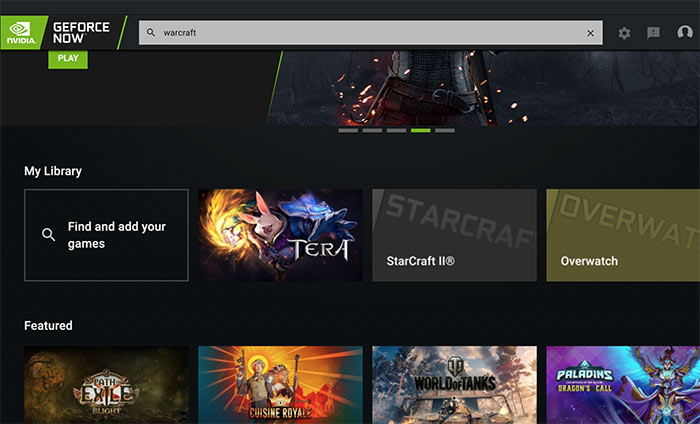This screenshot showcases the user interface of a website dedicated to video games, likely the NVIDIA GeForce Now platform. In the top left corner, we see the green NVIDIA logo, accompanied by the text "GeForce Now." Adjacent to this is a search bar with "Warcraft" entered into it. To the right, there are three icons: a gear representing settings, a comments button, and a profile photo button linking to the user's account.

Below this header section, a prominent banner displays a featured video game. Further down, the section labeled "My Library" appears with the prompt "Find and add your games." Listed here are games such as "Tera," "StarCraft II," and "Overwatch," indicating that they are part of the user's library.

Beneath the library section, there's a panel showcasing "Featured Games," which includes titles like "Path of Exile," "Cuisine Royale," "World of Tanks," "Paladins," and "Dragon Call." Each of these games is presented with a visually appealing background featuring their logos or key characters from the games, enhancing their appeal. Notably, "StarCraft II" and "Overwatch" simply display their names without additional imagery.